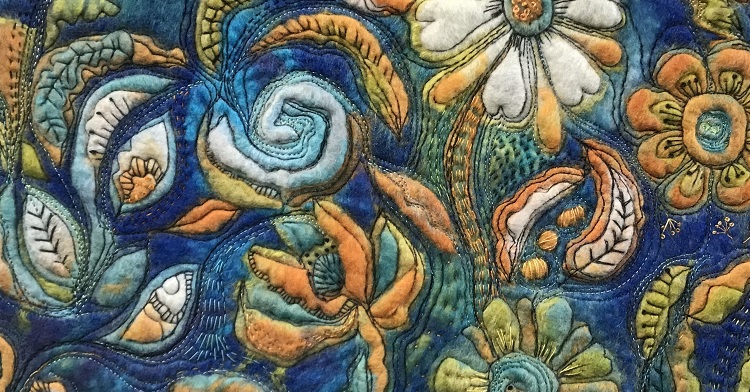This close-up photograph captures an intricately embroidered textile, likely a bed cover given the context. The vibrant fabric features a brilliant dark blue background adorned with elaborate stitched floral patterns in an array of colors. The rich design showcases flowers in shades of white, orange, blue, and green, interspersed with leaves in white, green, blue, and brown. Noteworthy elements include an orange flower with a blue center and surrounding yellow-green leaves to the right. On the left, there's a segmented golden-green vine topped with a large white flower and a blue-green petaled flower beneath it. Additionally, swirling blue and white designs and assorted floating flowers enhance the intricate composition. Detailed stitching in various colors—white, black, and blue—provides texture and depth, emphasizing the artistic, quilt-like quality of the piece.